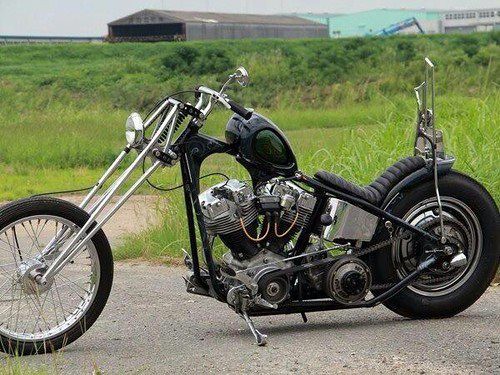The image depicts an outdoor setting featuring a motorcycle resting on its kickstand in the center of an asphalt road. The road is flanked by grassy fields on both sides. In the background, towards the top of the image, there are several buildings lined up, with a prominent gray, corrugated metal warehouse or barn-like structure. Another building nearby appears to have a mint green roof. A strip of sky, which is dark and dull yet bright, frames the top of the image. The motorcycle, black with silver metal poles and a kickstand, is positioned centrally on the asphalt, facing the left side towards the camera. This scene appears to be in the middle of the day, likely in a rural or farm-like environment.